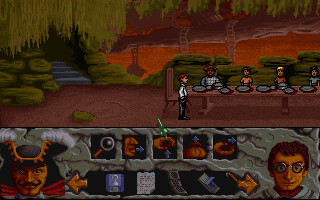This image is a screenshot from a video game, displaying a scene with intricate details that hint at a complex, adventure-filled storyline.

### Lower Section:
- **Bottom Left Corner**: An image of a pirate with a flamboyant curly mustache and a wild-eyed grin. The pirate is adorned with a blue hat, accentuated with gold trim and white feathers.
- **Bottom Right Corner**: A man with glasses sporting a slight smirk on the right side of his face. He has short brown hair and appears to be wearing a sweater (or perhaps a top with a collar).

### Center Section:
The center part of the screen is framed by what appears to be a rock-like interface. It contains five icons arranged horizontally:
1. **Magnifying Glass**: Possibly indicating a search or examine function.
2. **Person’s Face with a Blue Arrow**: This icon shows the face from the nose down to the chin with a blue arrow emerging from the mouth, likely indicating speech or interaction.
3. **Eyeball (or Hand) with Blue Arrow**: Initially described as an eyeball, this icon is actually a hand with a blue arrow pointing upward, suggesting an action to interact or grab.
4. **Bag with Blue Arrow**: A bag with a blue arrow above it, hinting at an inventory or storage feature.
5. **Hand (Palm Up) with Blue Arrow**: This icon appears to be a palm-up hand with a blue arrow pointing right, possibly indicating giving or offering.

A green push pin is conspicuously placed overlapping the interface at the third icon.

### Underneath the Icons:
- A black section features gold arrows on either side, likely for navigation. The segment includes:
  1. A floppy disk, indicating "Save."
  2. A piece of paper with written text, suggesting "Notes" or "Documents."
  3. An old-style cell phone, potentially for "Communication."
  4. A slightly ambiguous icon, resembling a book of matches.

### Upper Scene:
- **Foreground**: Displays an intricate cave structure with descending stairs and a backdrop of lush trees, especially a type with hanging branches reminiscent of an umbrella tree. Rocks are intricately piled, enhancing the natural setting.
- **Background**: Highlights a red-orange hue, illuminating a distant floating island with stairs leading to a tree branch, and two rope ladders suggesting an upward passage to a treehouse.
- **Inhabitants**: 
  - A man in a white shirt and black pants stands by a long table, positioned at its head.
  - Across the table sit several characters: A man in a red hat with dark skin, wearing a white shirt; a woman with short hair in an orange shirt; another woman with blonde hair in a darker orange shirt; and a woman with black hair wearing a gray shirt.
  - The table is set with two covered dishes and six plates, indicating a gathering or meeting. The beverages consumed are undefined.

The scene is richly detailed, combining elements of mystery, exploration, and interaction, all of which are crucial to progressing in the game.